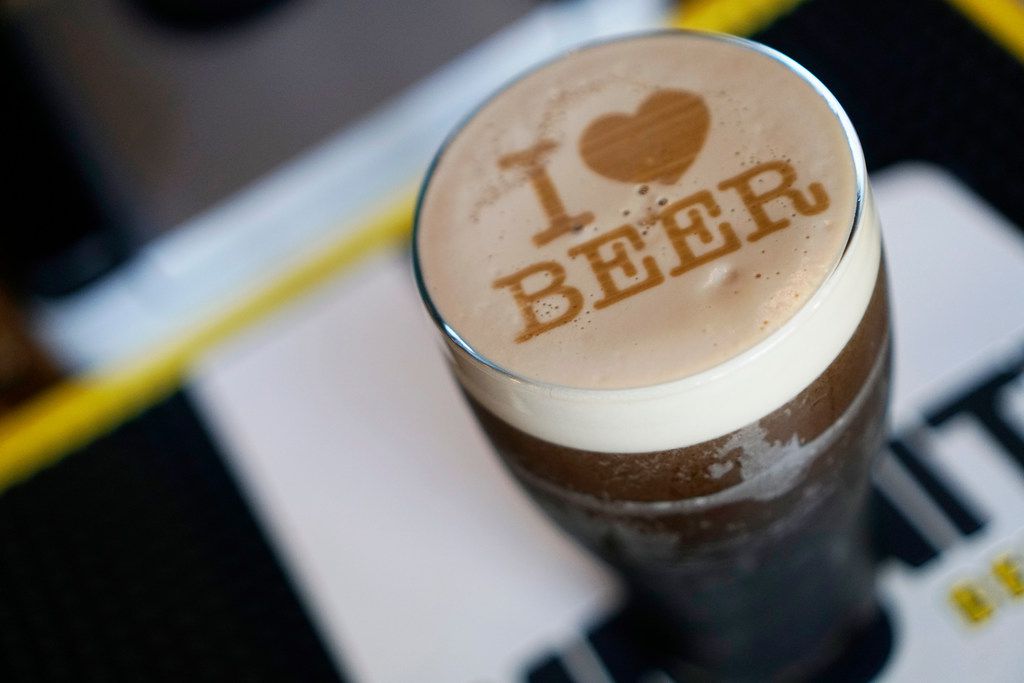The full-color, horizontally rectangular photograph, likely taken by a professional under artificial indoor lighting, carefully stages a clear glass of very dark brown beer, possibly a Guinness. The beer has a white, foamy head that reaches the rim of the glass. Intricately integrated into the foam is the message "I ❤️ BEER," with the heart represented by an image and the text styled in a clear, deliberate font, featuring golden-brown letters. The background appears out of focus, with some indistinct yellow lines, white spots, and black spots that could be napkins and straws, contributing to the overall composition without drawing attention away from the main subject.